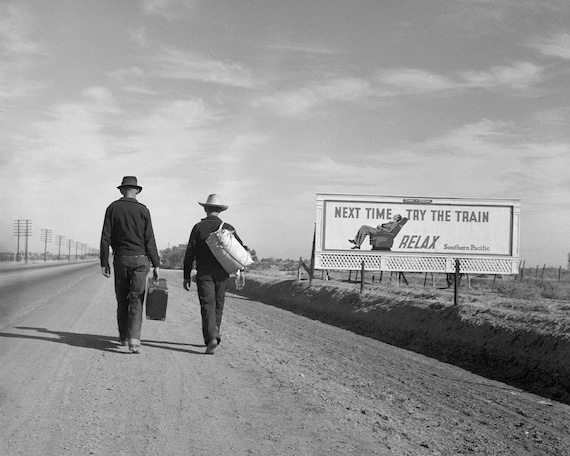This is a detailed black-and-white photograph capturing an evocative outdoor scene. The image is set under a mostly cloudy sky with areas of sunshine that cast shadows on the ground, indicating it is daytime. Dominating the foreground, two men walk away from the photographer down a dusty dirt road, which may have a partially paved section towards the extreme left. 

To the right side of the road, a large vintage billboard reads, "Next time try the train, relax," with "Southern Pacific" inscribed below. The billboard features a graphic of a man reclining comfortably with his legs outstretched, reinforcing the slogan’s suggestion. Both men are walking on the dirt shoulder next to the road, seemingly indifferent to the billboard's message.

On the left side of the photograph, a row of telephone or power poles stretches into the distance, adding depth and a sense of direction to the scene. The men are attired in period-specific clothing; the man on the left wears a 1920s-style hat, a black long-sleeve shirt, black pants, and carries a hard-shell suitcase in his right hand. The man on the right sports a cowboy hat, a black jacket, black pants, and a white duffel bag slung over his shoulder. The shadows cast by the men's figures confirm that the sun is shining despite the cloudy sky.

The photograph’s vintage feel, the attire of the men, and the design of the billboard suggest that it may have been taken in the 1950s, adding an element of historical context and irony as the weary travelers proceed on foot, evidently not "relaxing" as per the billboard’s advice.